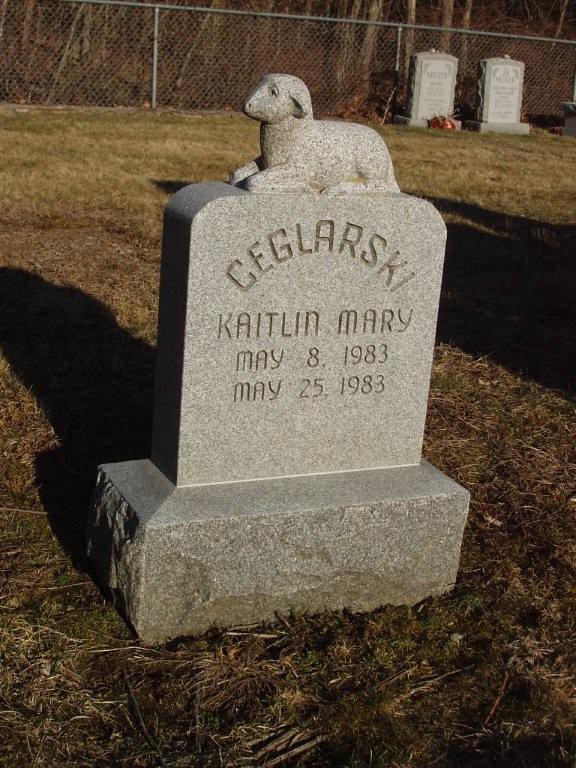The image depicts a grave in a cemetery, marked by a headstone made of gray stone. The headstone features a sculpted sheep lying on top, facing left, symbolizing the grave's occupant—a baby. The gravestone has a rectangular shape with the top two corners curved and rests on a lower platform. Inscribed on the stone is the surname "Ceglarski," spelled C-E-G-L-A-R-S-K-I, followed by "Caitlin Mary," with the dates "May 8, 1983 - May 25, 1983," indicating she lived for 17 days. The background reveals a fence and trees with two other tombstones, suggesting the season is either fall or winter, as the grass appears brown. The scene is tinged with a somber, late-evening light.